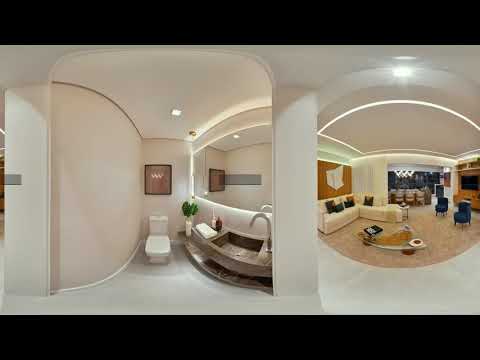The image is a wide, panoramic shot featuring two distinct sections: a bathroom on the left and a living room on the right, framed within a black border on the top and bottom. The bathroom is situated between two off-white square pillars and centers around a white toilet with the lid down, crowned by a pink piece of artwork above it. To the right of the toilet, a gray marble curved sink and a large, well-lit mirror add a modern touch.

The living room on the right side showcases a harmonious arrangement of furniture with an L-shaped beige couch adorned with several pillows on the left side, and two small dark blue velvet chairs positioned in front of a TV on a bright orange wooden cabinet on the right. A glass table with some indistinct objects adds to the room's contemporary feel.

The overall image is detailed and aesthetically pleasing, capturing a balanced, modern interior with varied colors including white, beige, brown, pink, blue, and orange. The panorama effect adds a unique curvature that visually separates and yet blends the distinct environments, providing a seamless transition between the bathroom and living room while maintaining a beautiful symmetry and a clear, crisp representation of both spaces.